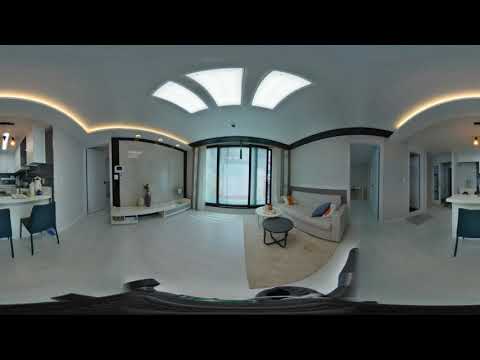The image showcases the interior of a modern, predominantly white room featuring a unique curvature due to the use of a panoramic or 360-degree lens. Centrally, straight ahead is a curved entranceway framed by a thick black border at the top and bottom, which accentuates the boundaries of the image. Above this entrance, three uniquely shaped skylights illuminate the area with natural light.

On the left side of the image, a display case and a desk with a chair are visible, adding to the room's functional aspects. Towards the middle of the space, a beige couch adorned with a black pillow is positioned on a tan, slightly dirty rug. In front of the couch sits a low, round black coffee table. The white counter, visible on both sides of the room due to the lens's curvature, is flanked by black chairs, adding a touch of contrast to the predominantly white decor.

On the right side of the image, you can discern part of a white countertop, leading to multiple doorways, and a glimpse of an open hallway. Both the left and right walls are highlighted by recessed lighting, further accentuating the clean, modern design. The ceiling, also painted white, is bordered by illuminated trim, enhancing the airy and spacious feel of the room. Various pieces of furniture, such as a white couch and low black tables, as well as small decorative objects and flowers, add character and charm to the minimalist decor.